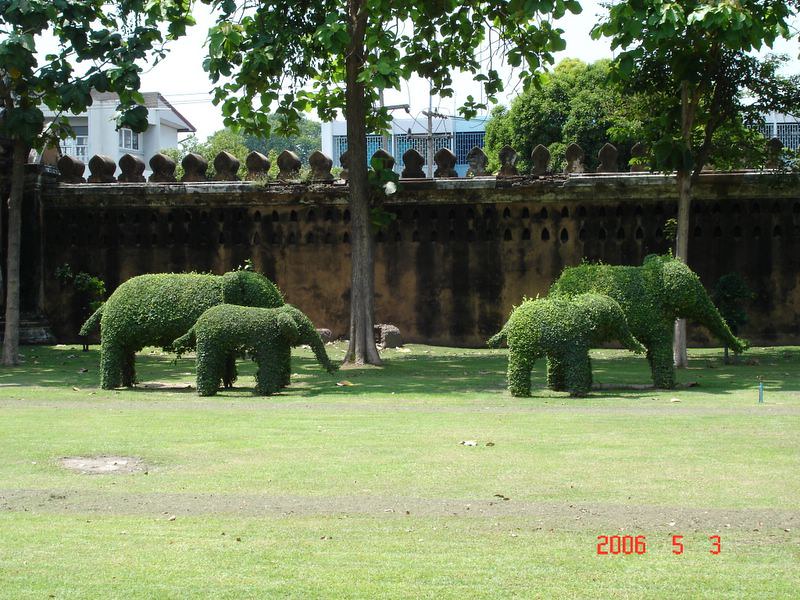This image captures an outdoor garden scene featuring four meticulously trimmed topiary elephants made from green hedges. The elephants are arranged with two pairs: one adult and one smaller elephant in the front towards the right, and another pair of differing sizes behind them. Each elephant is facing to the right. Surrounding this verdant display is a well-maintained grassy area with a few bare patches and three tall, slender trees with deciduous green leaves. A cement wall with crenellation details and a rounded pedestal borders the garden, and in the background, some buildings, including what appear to be a white house and a blue house, are visible. Red text in the bottom right corner of the image indicates the date: May 3rd, 2006.